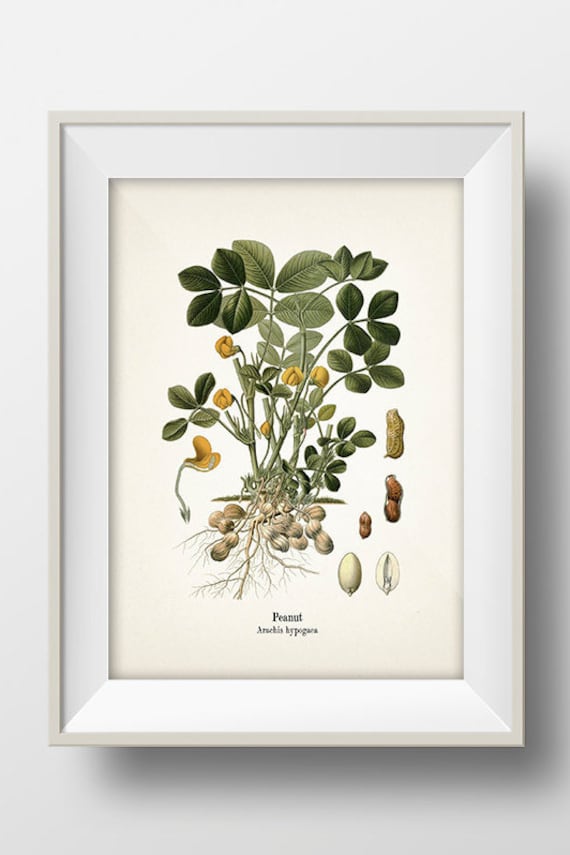The image depicts a detailed botanical illustration of a peanut plant framed in a white picture frame, mounted against a white wall. The print features a creamy white background that adds a vintage touch. The focal point is the meticulously drawn peanut plant showcasing its various parts, from the roots at the bottom to the green foliage and yellowish flowers at the top. Accompanying the main illustration are close-up drawings on the right, depicting the different stages of peanut development. These range from initial white bulbs to fully matured peanuts in darker shades of brown. The label "peanut" is prominently displayed beneath the main plant image, along with a Latin name that is not fully legible. The white frame casts a subtle shadow to the right, suggesting natural light. This botanical print has the appearance of an art piece commonly found on platforms like Etsy.